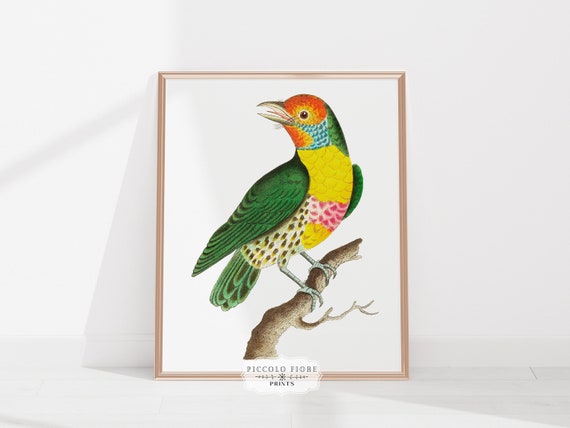The image depicts a vibrant and colorful painting of a bird, enclosed in a metal frame, leaning against a white wall and casting a shadow. The bird, which appears to be a toucan or parrot, is composed of an array of stunning colors: its head is a mix of orange and yellow, it has blue and green feathers, its breast features yellow, pink, brown, and white feathers, and its wings and tail are primarily green. The bird is perched on a brown branch with both feet and has its beak open, revealing its tongue, as if it is making a sound or eating something. The artwork bears the watermark "Piccolo Fiore Prince," indicating the artist.